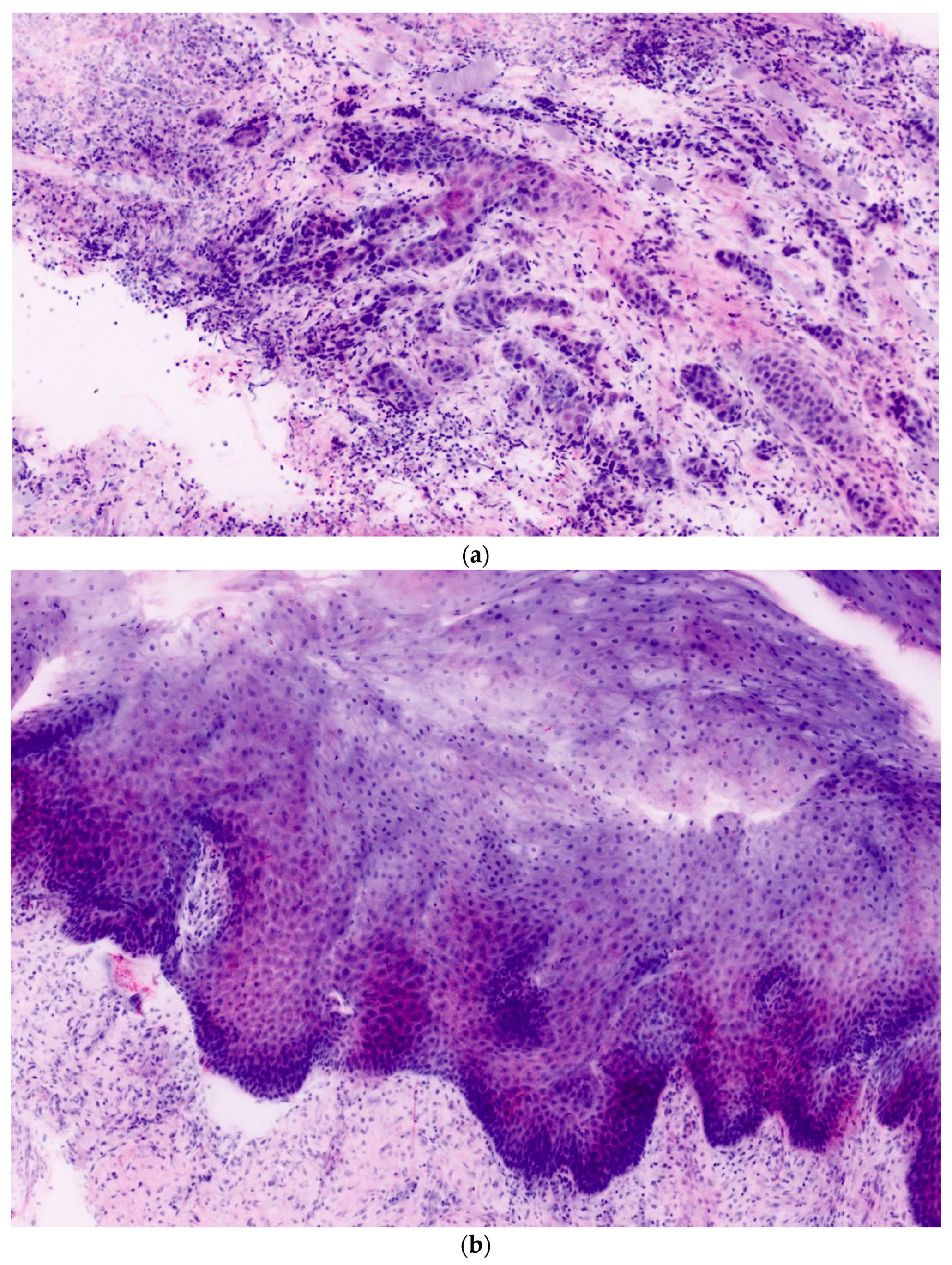The image consists of two microscopic views, each occupying half the picture. The top half, labeled "lowercase a," displays a specimen stained with various hues of purple, scattered against a white background. The specks or dots are dispersed throughout the image, reminiscent of bacteria or microorganisms under a microscope. In contrast, the bottom half, labeled "lowercase b," shows a similar microscopic view but with a distinct difference: a denser concentration of dark purple specks forming what appears to be a wave-like or lumped mass that spans the width of the image, with lighter areas towards the edges. Both images exhibit the same sized specks, differing primarily in their distribution and pattern.